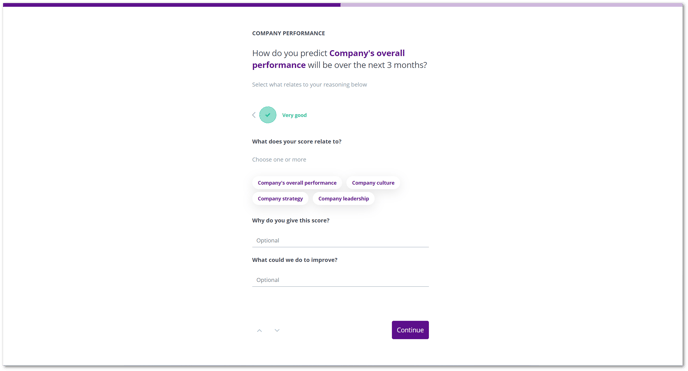This screenshot is from a website or software interface featuring a survey form evaluating company performance. At the top, a gradient purple bar transitions from dark purple on the left to light purple on the right. Below this bar, the section header "Company Performance" appears in black text. The survey question asks, "How do you predict the company's overall performance will be over the next three months?" with the phrase "company's overall performance" highlighted in purple. 

Following the question, additional instructions in black text read, "Select what relates to your reasoning below." The selected option "Very Good" is highlighted in teal. The next prompt states, "What does your score relate to? Choose one or more," and provides options in purple ovals: "company's overall performance," "company culture," "company strategy," and "company leadership."

Further down, another question in black asks, "Why do you give this score?" followed by an optional text input bar for responses. A subsequent prompt asks, "What could we do to improve?" with another optional text input field. 

At the bottom of the screenshot, a purple rectangle with white letters offers a "Continue" button. This summary encapsulates the entire layout of the survey page.